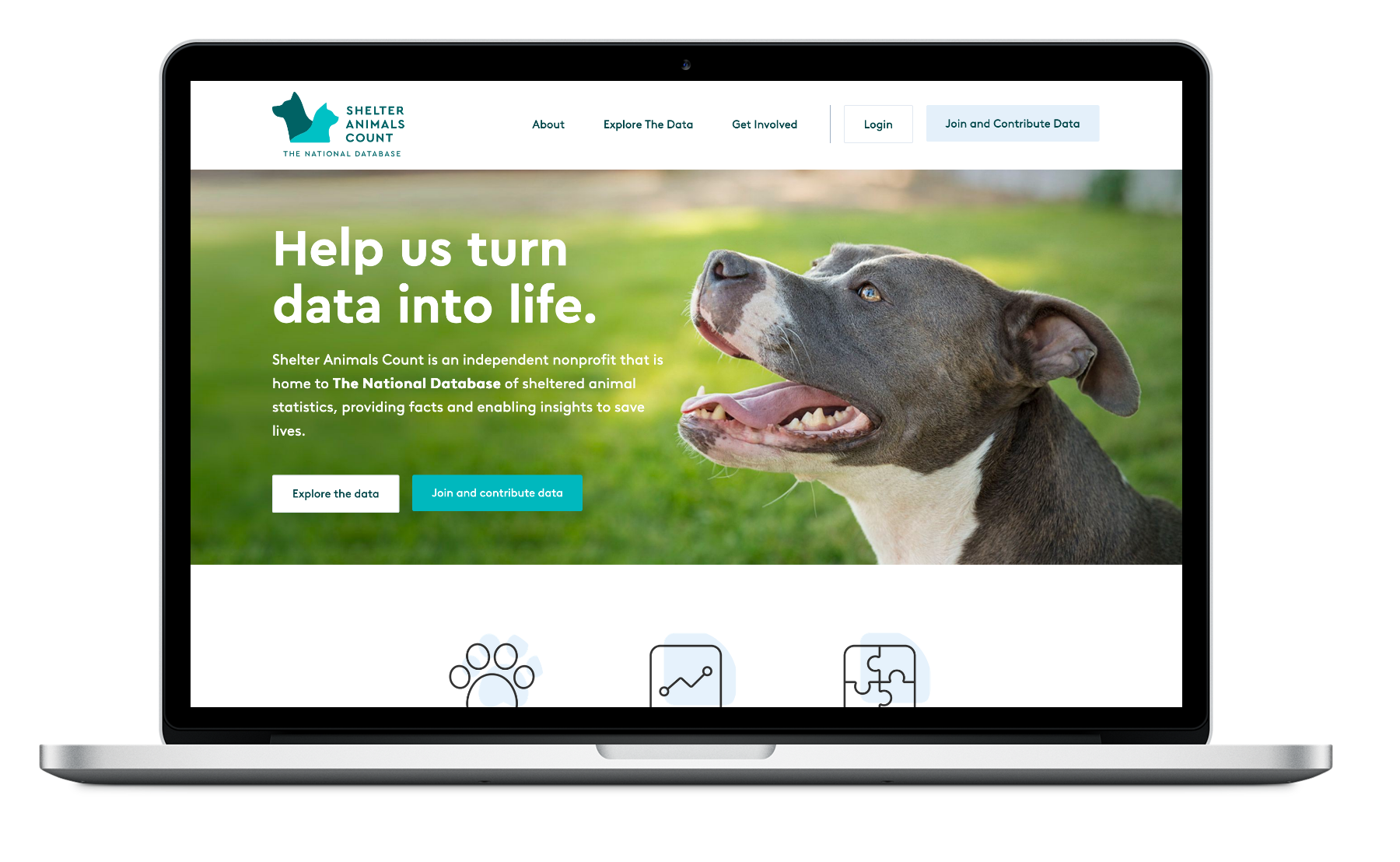The image features a silver shelf centered on a white background, holding an iPad. The iPad's screen, with a black perimeter, displays information about shelter animals under a banner titled "Shelter Animals Count." To the left of the banner is a dark and light blue silhouette of a dog, next to dark blue uppercase text that reads "SHELTER ANIMALS COUNT." To the right, there are navigational options: "About," "Explore the Data," "Get Involved," and buttons for "Login" and "Join and Contribute Data" (the latter shaded light blue).

At the center of the screen is a vibrant photograph of a dog, predominantly white and dark brown, looking to the left. The dog’s mouth is open, revealing a big pink tongue, sharp teeth, and pink gums, with ears pointed backward. To the left of the dog is a prominent message in large white font: "Help Us Turn Data Into Life." Below that, in smaller white font, a brief description states, "Shelter Animals Count is an independent nonprofit that is home to the National Database of Sheltered Animal Statistics, providing facts and enabling insights to save lives."

At the bottom of the screen, a white rectangular banner contains two buttons: one white with dark green text reading "Explore the Data," and the other blue with white text reading "Join and Contribute Data." Below this banner, a separate white rectangular area features three icons: a paw print, a cell phone, and a jigsaw puzzle piece, each symbolizing different functionalities or sections.